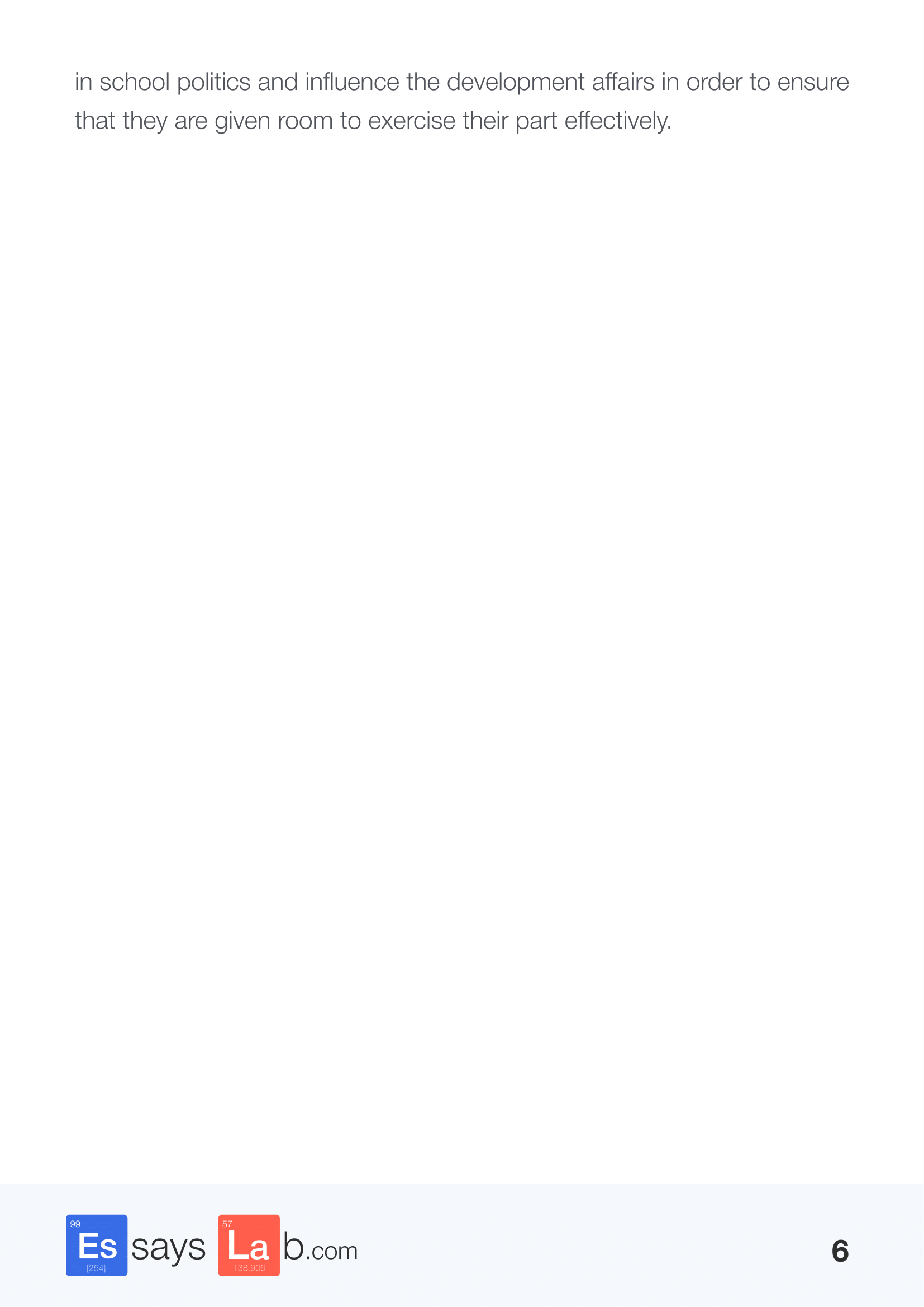This image displays a minimalist poster primarily consisting of a large expanse of white space. At the top, there is text that reads: "In school politics and influence the development affairs in order to ensure that they are given room to exercise their part effectively." The middle portion of the poster is entirely blank, emphasizing the simplicity of the design. At the bottom of the poster, the website "essayslab.com" is prominently featured; the "ES" in "essay" is enclosed in a blue square, while the "LA" in "lab" is enclosed in a red square, providing a pop of color against the stark white background. In the bottom right corner of the poster, the number "6" is visible, possibly indicating a version or edition.